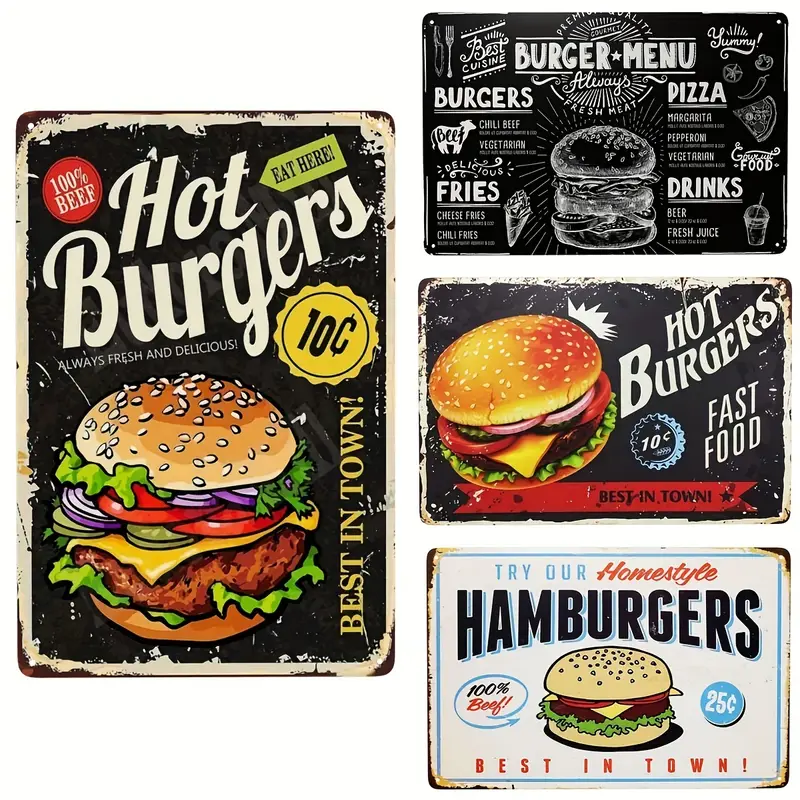The image depicts a collection of nostalgic advertisement posters with a burger theme, set against a white background. The first poster on the left, a vertically oriented black rectangle with a white trim, features a worn, chipped appearance and reads: "100% beef, eat here, hot burgers, 10 cents, always fresh and delicious, best in town." It is adorned with a vibrant image of a classic hamburger, complete with lettuce, cheese, tomato, onions, and a sesame seed bun. To its right, three horizontal rectangles are arranged vertically. The topmost sign, another black rectangular poster, is titled "Burger Menu" and lists various food items including burgers, chili beef, vegetarian, delicious fries, cheese fries, chili fries, pizza (margarita, pepperoni, vegetarian), along with drinks such as beer and fresh juice. The middle sign, also black, boldly declares "Hot Burgers, Fast Food, 10 cents, best in town," accompanied by an enticing image of a hamburger. The bottom sign, a white rectangle, encourages customers to "Try our homestyle hamburgers, 100% beef, 25 cents, best in town." Each sign exudes a retro charm, highlighting the affordability and appeal of the burgers they advertise.